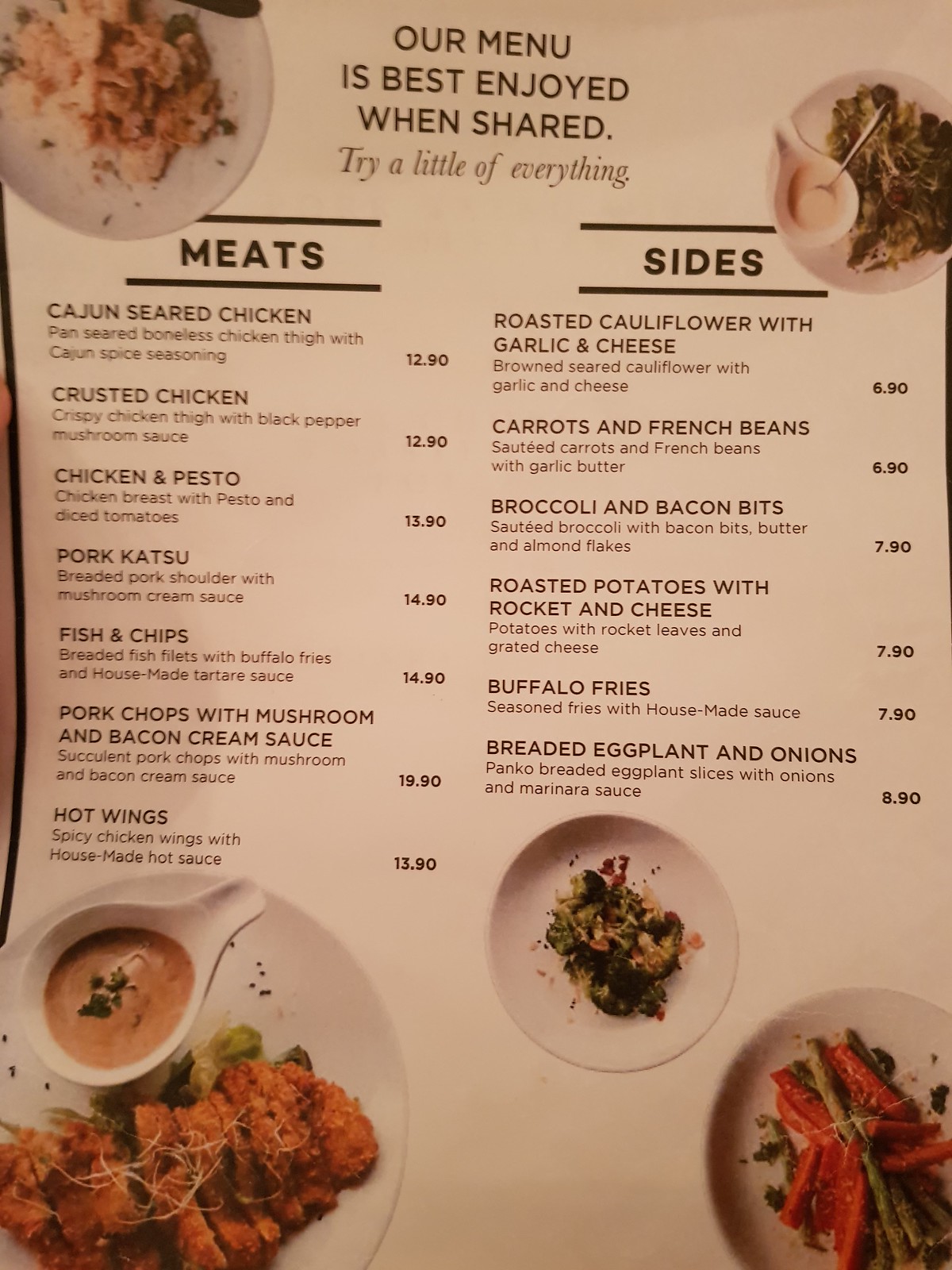This top-down photograph captures a rustic restaurant menu, intricately detailed with visual plate presentations and item descriptions in two neat columns. The menu is captured against a white background, giving it a clean and appetizing look.

The layout features five different food plates, strategically placed for visual appeal: two in the top corners, two in the bottom corners, and a smaller plate in the center. Each plate showcases a tantalizing display of food, providing a sneak peek into the menu offerings. The top left plate features creamy mashed potatoes, while the top right plate displays vibrant cooked greens—broccoli or collard greens—accompanied by a ladle of white sauce. The bottom left plate presents a breaded cutlet-style meat, sliced and laid atop fresh greens, paired with another ivory-colored sauce in a ladle. Adjacent to this, another plate of greens contributes to the colorful array. The bottom right plate rounds off the selection with a medley of green asparagus and orange carrot sticks.

The menu itself is printed in sleek black text on a pristine white background. At the very top, inviting text reads: "Our menu is best enjoyed when shared. Try a little of everything." This sets the tone for a communal dining experience.

The left column is devoted to "Meats," listing seven enticing entries:

1. Cajun Seared Chicken
2. Crusted Chicken
3. Chicken and Pesto
4. Pork Katsu
5. Fish and Chips
6. Pork Chops with Mushroom and Bacon Cream Sauce
7. Hot Wings

The right column is labeled "Sides" and details six delectable options:

1. Roasted Cauliflower with Garlic and Cheese
2. Carrots and French Beans
3. Broccoli and Bacon Bits
4. Roasted Potatoes with Rocket and Cheese
5. Buffalo Fries
6. Breaded Eggplant and Onions

Each item is paired with a corresponding price, meticulously listed to the side, allowing for easy reference.

Overall, the image and menu work harmoniously to tempt and intrigue with their inviting presentation and diverse offerings.